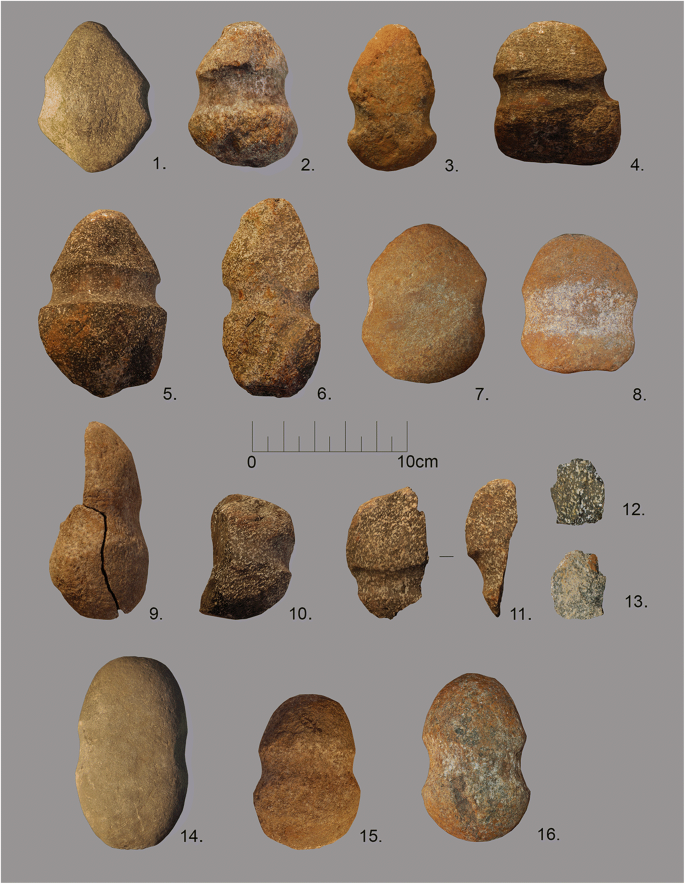This image exhibits 16 distinct, prehistoric-looking rocks meticulously arranged on a gray background. Each rock bears a unique label from 1 to 16, starting from the top left corner. Number 1, positioned in the top-left, is a tan rock with black stripes, resembling a dull arrowhead. Number 2 appears even more worn, hinting at use as a tool with visible ridges. Number 3, similar in function, resembles an Indian arrowhead. The rocks vary in shape, some more rounded and natural-looking, while others appear intentionally carved, clearly shaped by human hands.

Predominantly, the rocks exhibit shades of reddish, brown, tan, and gray. They are organized into rows: four in the first, four in the second, six in the third, and three in the last. Notably, many of the rocks feature pointed tips and chipped middle sections, suggesting they could be ancient arrowheads or tools. A ruler in the image measures up to 10 centimeters, revealing that most rocks are close to this size, although a few, like numbers 12 and 13 in the third row, are distinctly smaller. This detailed arrangement and presentation hint at the rocks' historical and archeological significance.